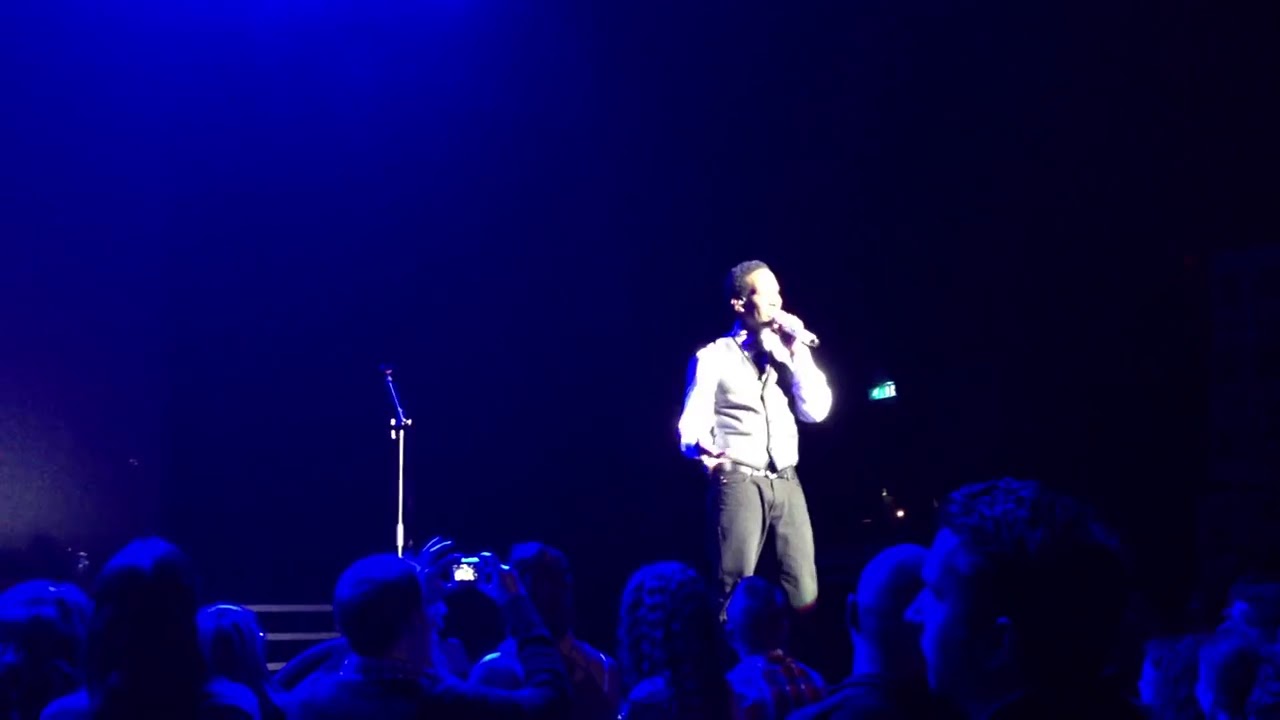The image depicts a man performing at what seems to be a concert, perhaps held in a church, as indicated by the presence of what might be an exit sign in the blurry background. The performer is slightly out of focus and overexposed, likely due to a spotlight shining on him, making it challenging to distinguish specific details of his attire; he appears to be wearing a light-colored long-sleeve button-down shirt and dark pants, possibly gray or brown. Holding a microphone close to his face with his left hand, his right hand rests by his side. Positioned on the left side of the stage, a silver microphone stand is visible behind him. The audience, captured from behind, is bathed in a deep indigo blue light emanating from both the background and above, illuminating several rows of concertgoers whose heads and side profiles are discernible. Additionally, one person near the front appears to be taking a picture with a phone camera, adding to the dynamic atmosphere of the scene.